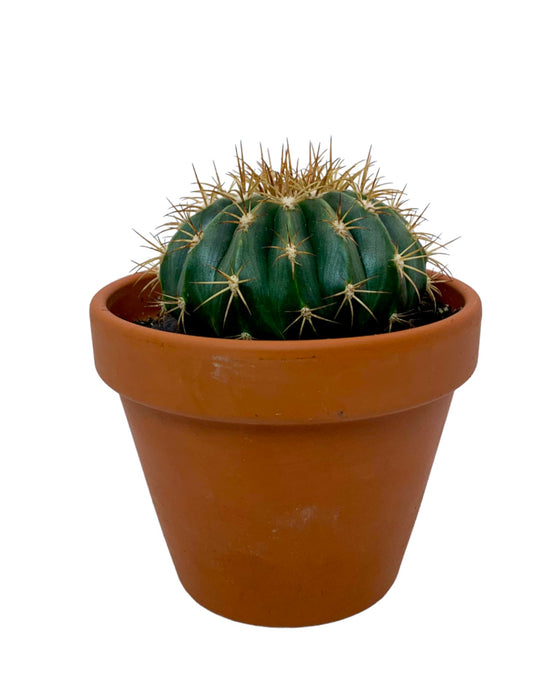The image captures a close-up view of a small, round, pumpkin-shaped cactus planted in an older, discolored, terracotta clay pot. The cactus is dark green with distinctive ribs, resembling those of a pumpkin, and covered with tan-colored and light brown spikes that are sparse on the sides but become denser towards the top. The pot itself is cone-shaped with an extruded lip and filled with dark, recently watered soil. Set against a pure white background and placed on a white surface, both the pot and cactus are centered in the image, creating a minimalist and focused composition. The angle of the photograph allows a clear view of the soil inside the pot, contributing to the overall rustic and natural aesthetic.